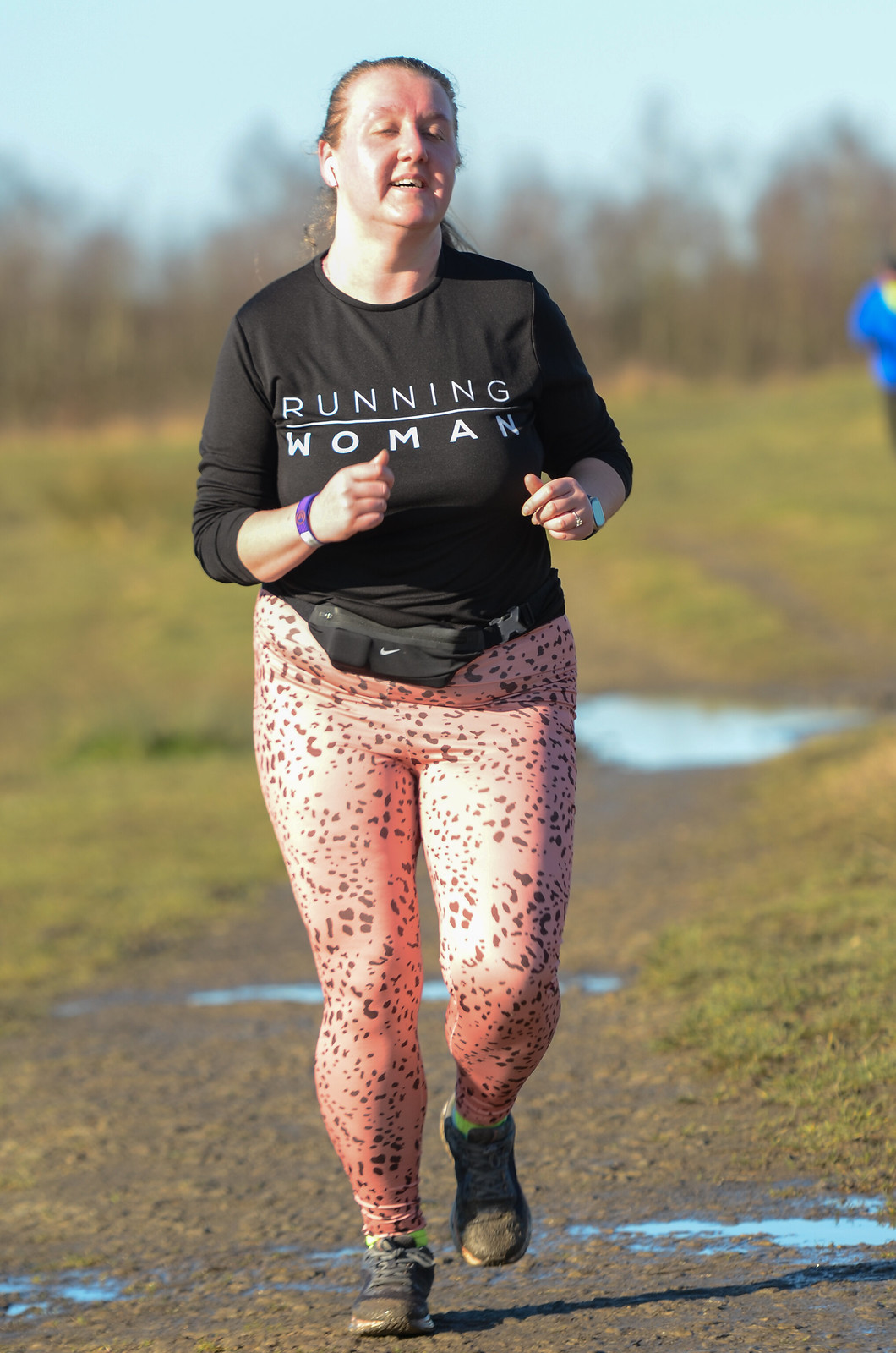The photograph captures a white woman with blondish-brown hair jogging outdoors on a wet, muddy dirt trail after a recent rainfall. She is slightly heavyset and is wearing a black, long-sleeved running shirt with the text "Running Woman" in white letters. A purple wristband adorns her right wrist, while her left wrist features either a white wristband or wristwatch. Around her waist, she sports a black Nike fanny pack with a white logo. Her lower body is clad in pinkish, cheetah-print spandex pants with black spots. Her shoes are black with white laces and some green accents, visibly muddied from the trail. Surrounding her, the trail is punctuated by several puddles, flanked by green and yellow grass, and bare, brown trees can be seen in the distant background under a blue and white sky. In the far right background, a person in a blue shirt and dark pants is visible.